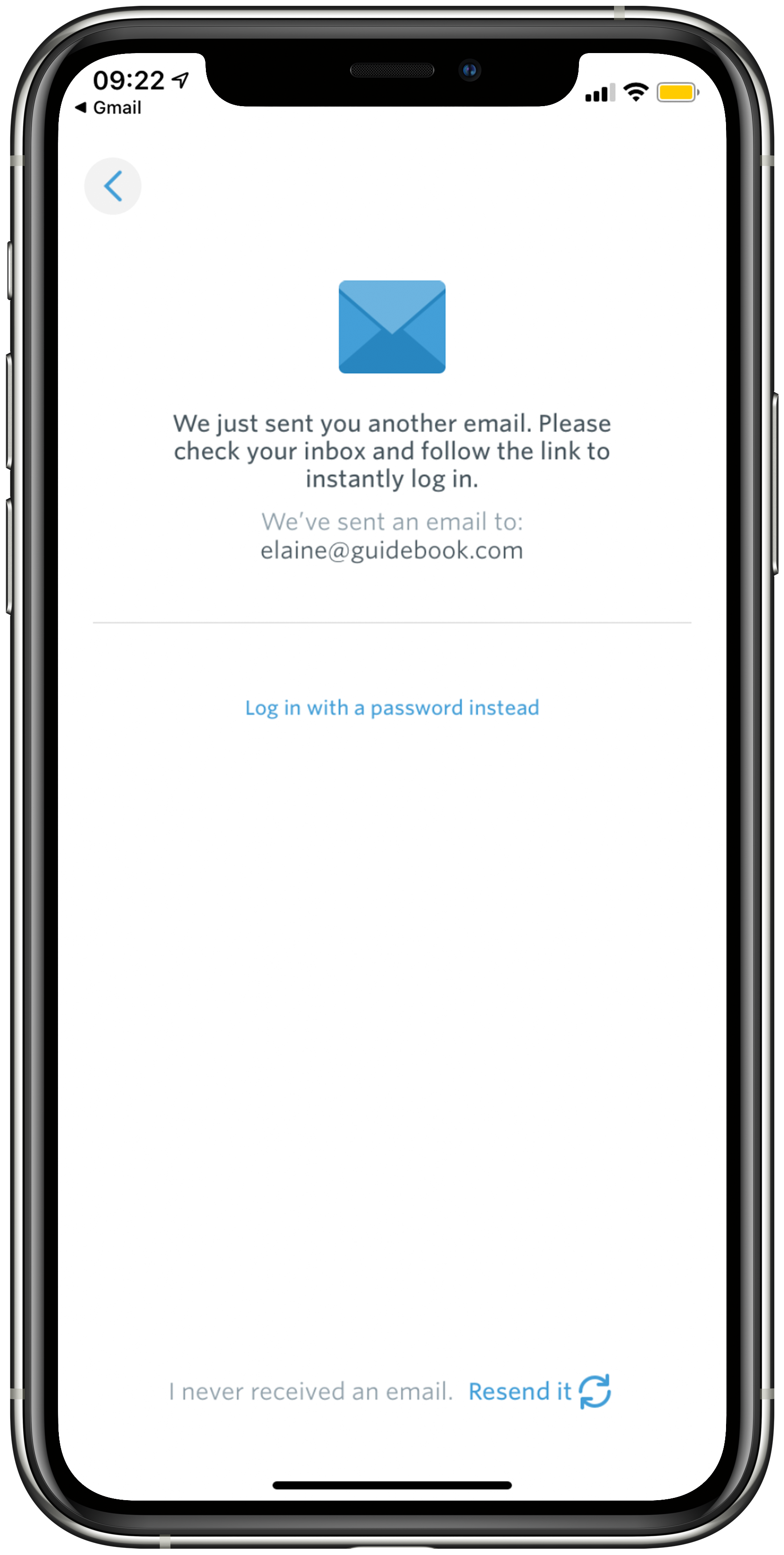The image depicts a mail application interface on a smartphone. At the top center, there is a blue envelope icon with varying shades of blue. Below this, on a white background, black text reads: "We just sent you another email. Please check your inbox and follow the link to instantly log in. We've sent an email to elaine@guidebook.com." Beneath this, there is a clickable blue text stating, "Log in with a password instead." Further down, gray text says, "I never received an email," accompanied by a blue button on the bottom right corner labeled "Resend it," featuring a circular icon of blue circulating arrows. On the top left, there is a back button, represented by a left-pointing arrow inside a gray shaded circle. The overall background of the interface is white, and elements of the smartphone's frame are visible at the bottom of the page, indicating that this is indeed a screenshot from a mobile device.